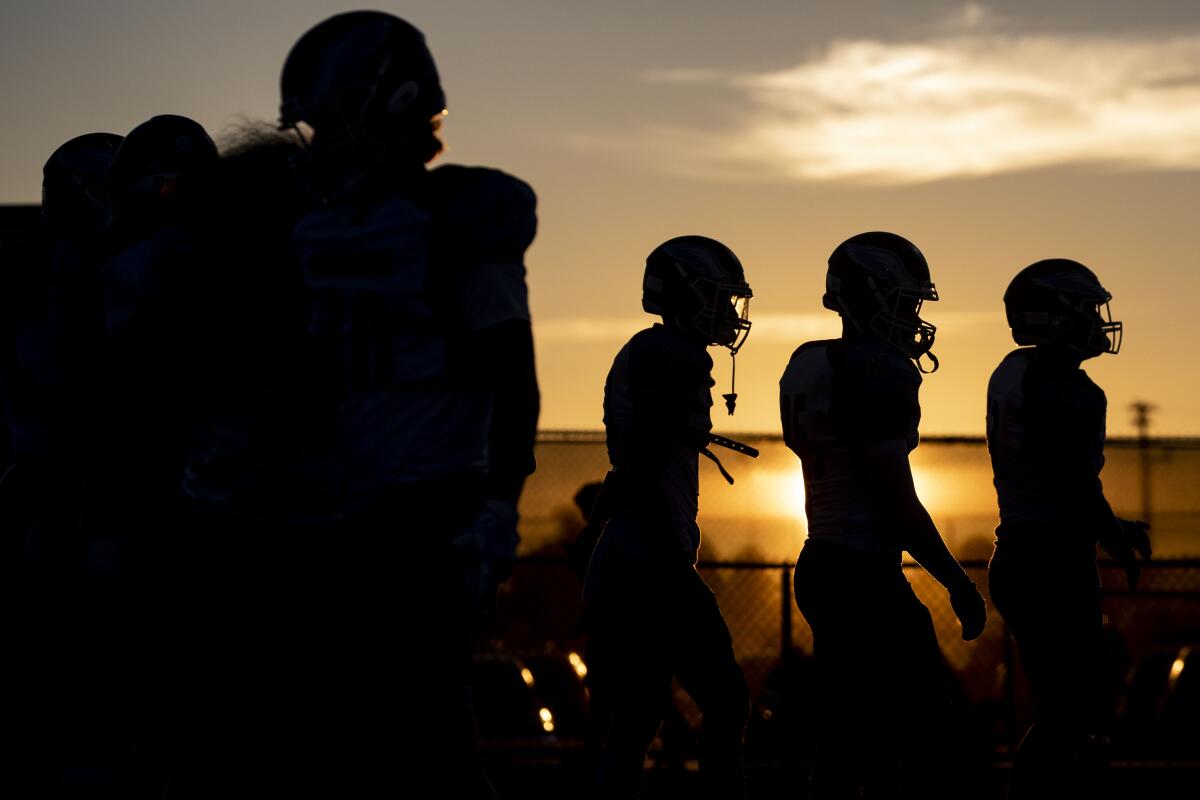This angled photograph captures the dramatic silhouettes of football players walking along a field, bathed in the warm glow of a setting sun. On the right side of the image are three players, clearly outlined by their helmets, face guards, and large shoulder pads with straps. The player in the forefront has a mouth guard dangling from the helmet. Further back are additional players whose helmet crowns and shoulder pads are faintly visible. The sky above them is a dark gray with accents of orange and yellow from the sunset, and a wispy white cloud hovers in the top right corner. In the background, a tall metal fence stands silhouetted against the fading light, while a smaller, closer fence is illuminated by the sun's golden rays. A large light post is also visible on the right side, adding to the composition's layered depth. The overall scene is imbued with a sense of tranquility and transition, as the day gives way to evening.